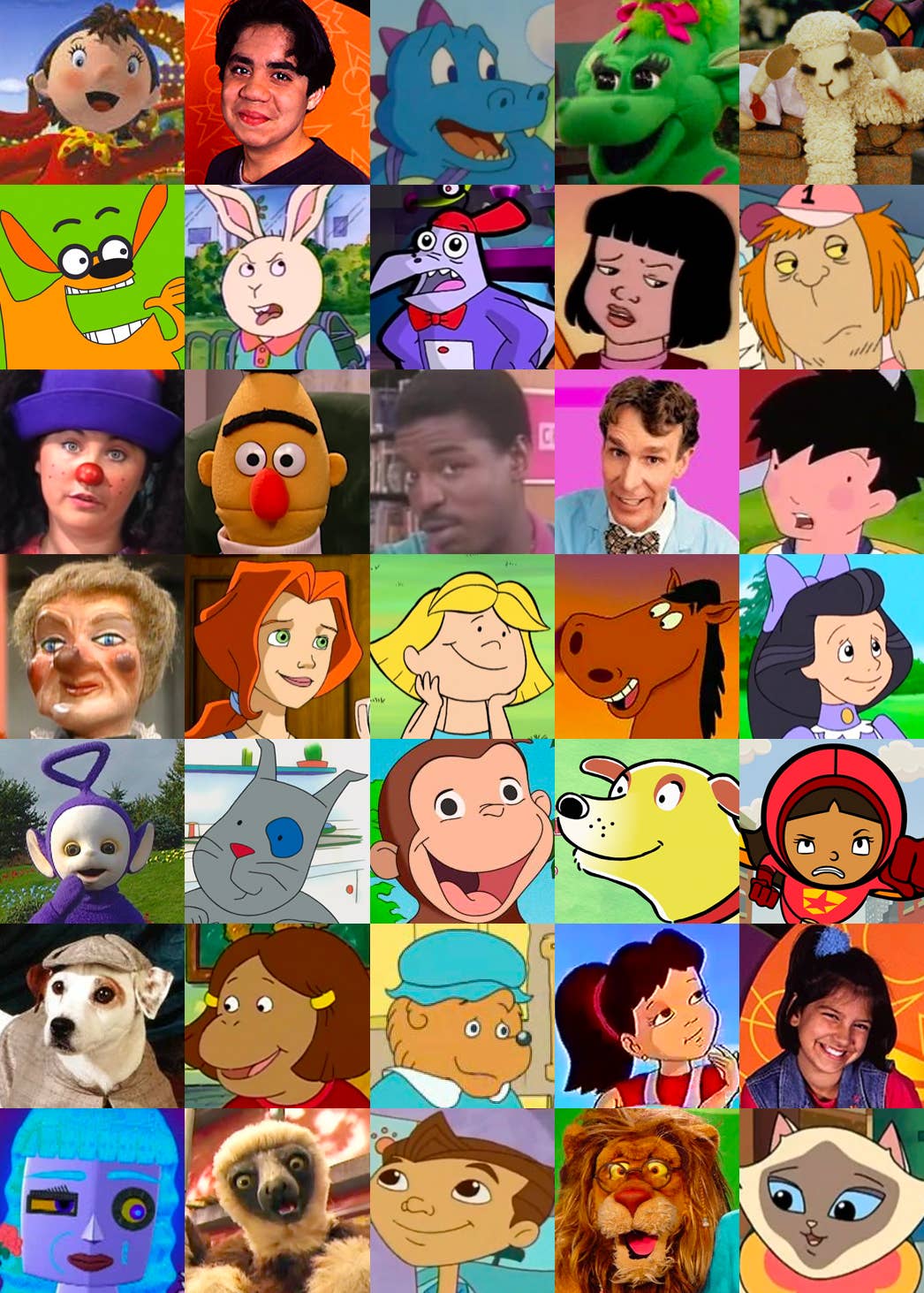In this vibrant and dynamic image, we observe a grid composed of 35 square-shaped pictures, meticulously arranged in 7 rows and 5 columns. Each square features a distinct face, either of an animated cartoon character or a real person, creating a diverse mosaic of expressions and styles.

The top-left square showcases the cheerful cartoon character Noddy, easily identifiable with his distinctive hat and smile. Adjacent to Noddy, moving rightward, is a square that contains a real photograph of a man. His facial features are clearly visible, along with a portion of his shoulder, set against a striking orange background. Continuing to the right, the subsequent square depicts a blue dragon cartoon character, adding a whimsical touch to the array.

Each square bursts with color, contributing to the overall vivacious ambiance of the image. The combination of vivid illustrations and realistic photographs engenders an engaging visual interplay that captivates the eye. The consistency in the layout—each face framed within an equally sized square—provides a harmonious structure, allowing the viewer to appreciate both the individual elements and the collective composition.